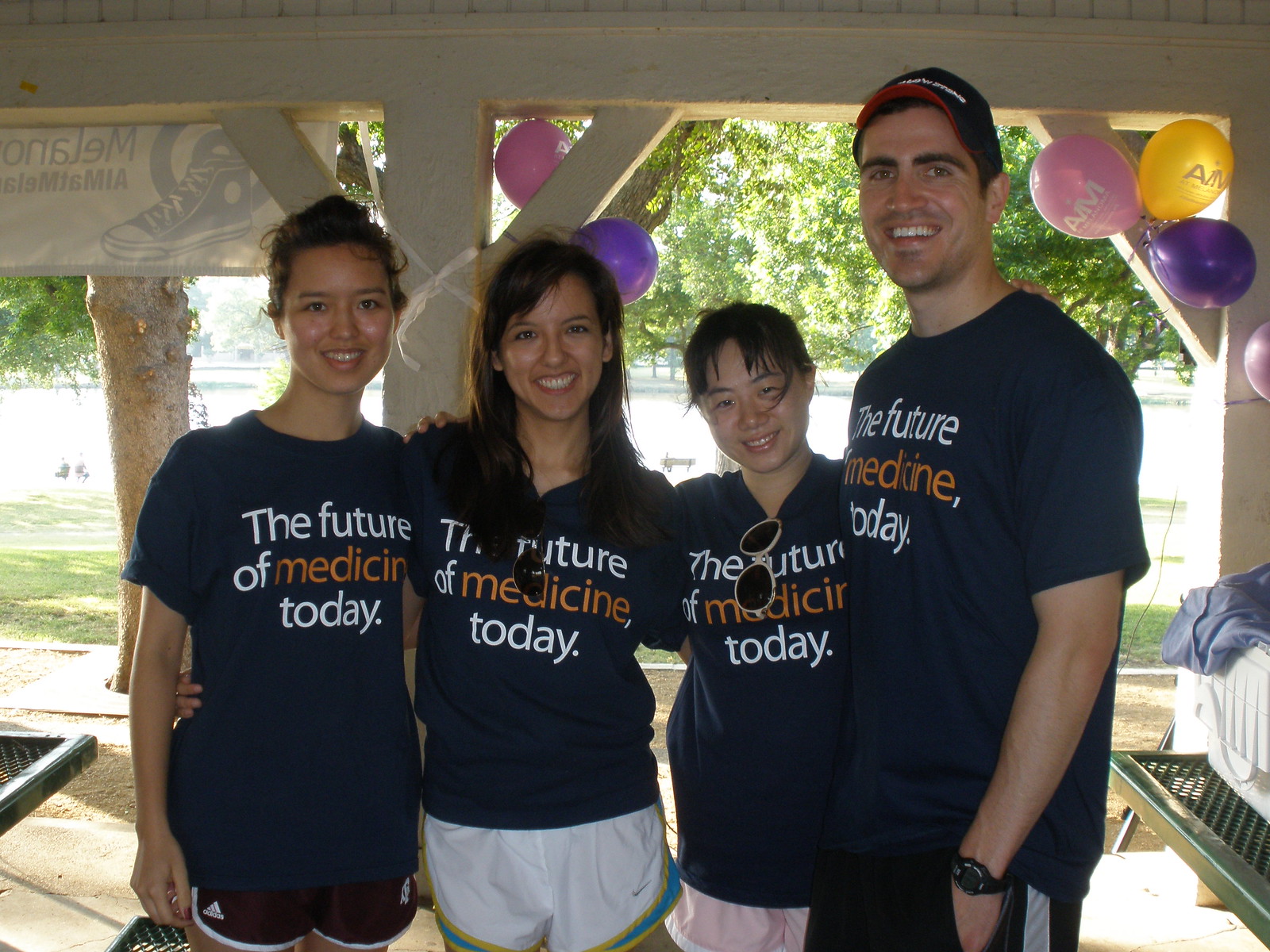The photograph captures a cheerful family of four at a party, all dressed in matching navy blue t-shirts emblazoned with the slogan "The Future of Medicine Today." The text on the shirts is mostly white, with the word "Medicine" standing out in an orangish hue. The family consists of three women and one man. On the left is a young girl, followed by a woman who appears to be in her 30s or 40s. Next to her stands another young girl, and on the far right is the man, presumably the father, who is middle-aged and wearing a hat and a watch. Two of the women have sunglasses clipped to their shirts. They are standing in a white pavilion adorned with festive pink, purple, and yellow balloons, with the bright sunlight and lush green trees visible through the background, indicating it's a beautiful day outside.